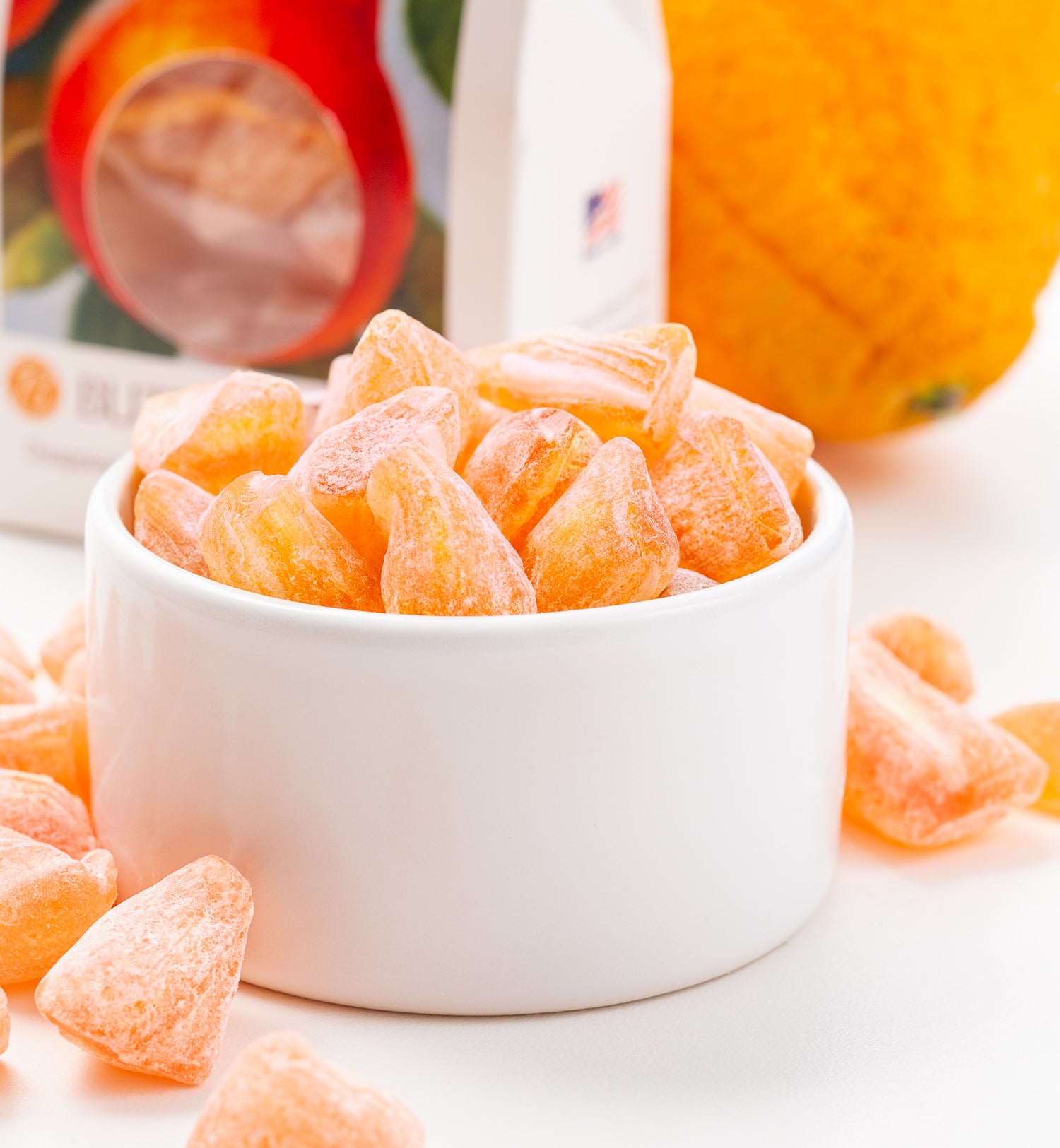The image depicts a bright and detailed tabletop scene, likely set in a kitchen. At the center, there is a pristine white, flat-bottomed, slightly raised porcelain bowl filled with an assortment of round and triangular orange-colored candies or gummies. These gummies are dusted with a light, powdery substance that gives them a sugar-coated appearance. Behind the bowl, slightly to the right, there is an actual orange fruit, adding a touch of realism to the scene. Further in the background, also to the right, is a box with a striking red, orange, and white design, suggesting packaging for the candies. Additionally, there are hints of a white bag with American flag motifs and a darker red, possibly blood orange fruit accompanied by green leaves. The entire setup rests on a light-colored, white tabletop, and the photograph’s focus brings sharp clarity to the bowl and candies while slightly blurring the background elements, enhancing the overall aesthetic and drawing attention to the featured treats. This composition suggests a professionally taken photograph, potentially for an advertisement or a culinary showcase.